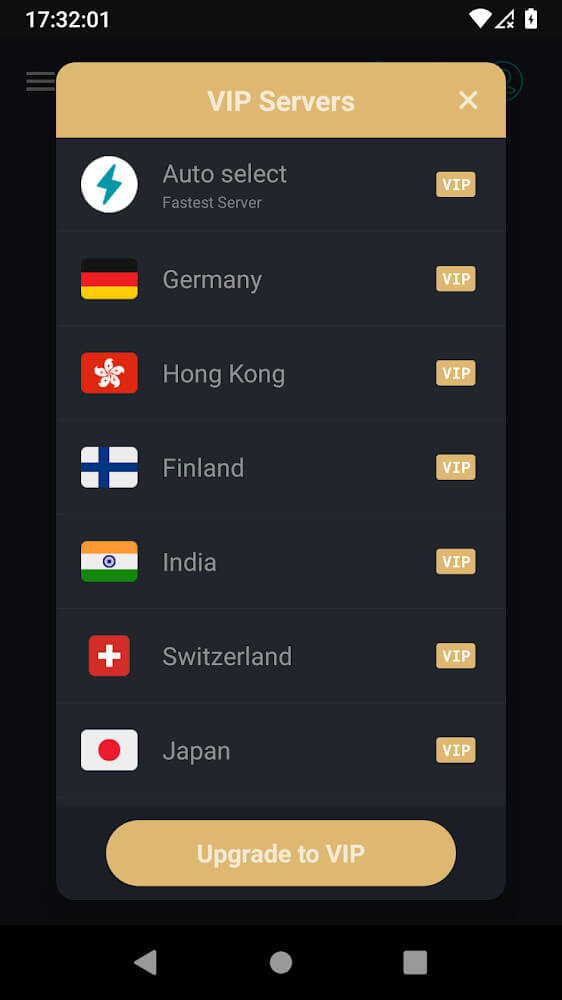The image displays a digital interface with a prominent black header at the top. In the top-left corner, the header features a timestamp, reading "17:32:01." Moving rightward within the header, icons depict the Wi-Fi signal status, which is active, the mobile signal status, showing no reception bars, and the battery level, which appears to be relatively full.

Below this primary black header is a slightly lighter black rectangle with rounded corners, serving as a sub-header. This sub-header reads "VIP servers" and has a close icon (X) on its far right. Below this sub-header is a list of server options.

The first item on the list is "Auto Select," which is accompanied by a description stating "Fastest server"; a VIP button is situated to the right of this item. The following items in the list are various country servers, each denoted by the respective national flag and a VIP button on the right side. The countries listed are:

1. Germany, with an icon of the German flag.
2. Hong Kong, with an icon of the Hong Kong flag.
3. Finland, with an icon of the Finnish flag.
4. India, with an icon of the Indian flag.
5. Switzerland, with an icon of the Swiss flag.
6. Japan, with an icon of the Japanese flag.

At the bottom of the interface, a footer section encourages users to "Upgrade to VIP." Below this invitation, there are three distinct icons, though their specific details are not described in the text provided.